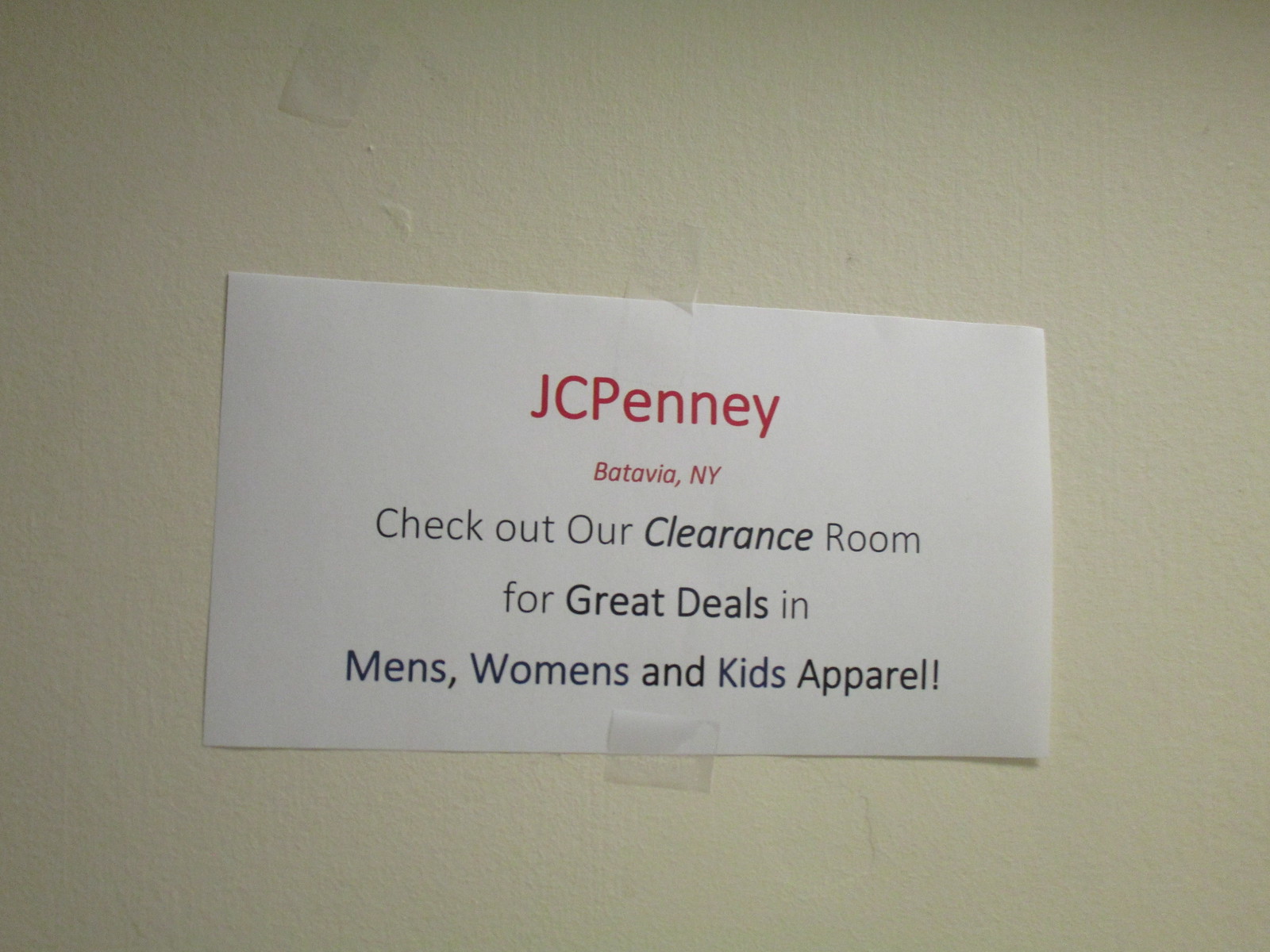A piece of paper is taped to a white, cemented wall, bearing some visible marks. The paper displays red text that prominently reads "JCPenney" at the top in bold letters. Below it, in a smaller font, it specifies the location as "Batavia, New York." The message on the paper invites customers to "Check out our clearance room for great deals in men's, women's, and kids' apparel." This promotional note, repeated more than once, is affixed to the wall, serving as an eye-catching announcement for the store's clearance sale.